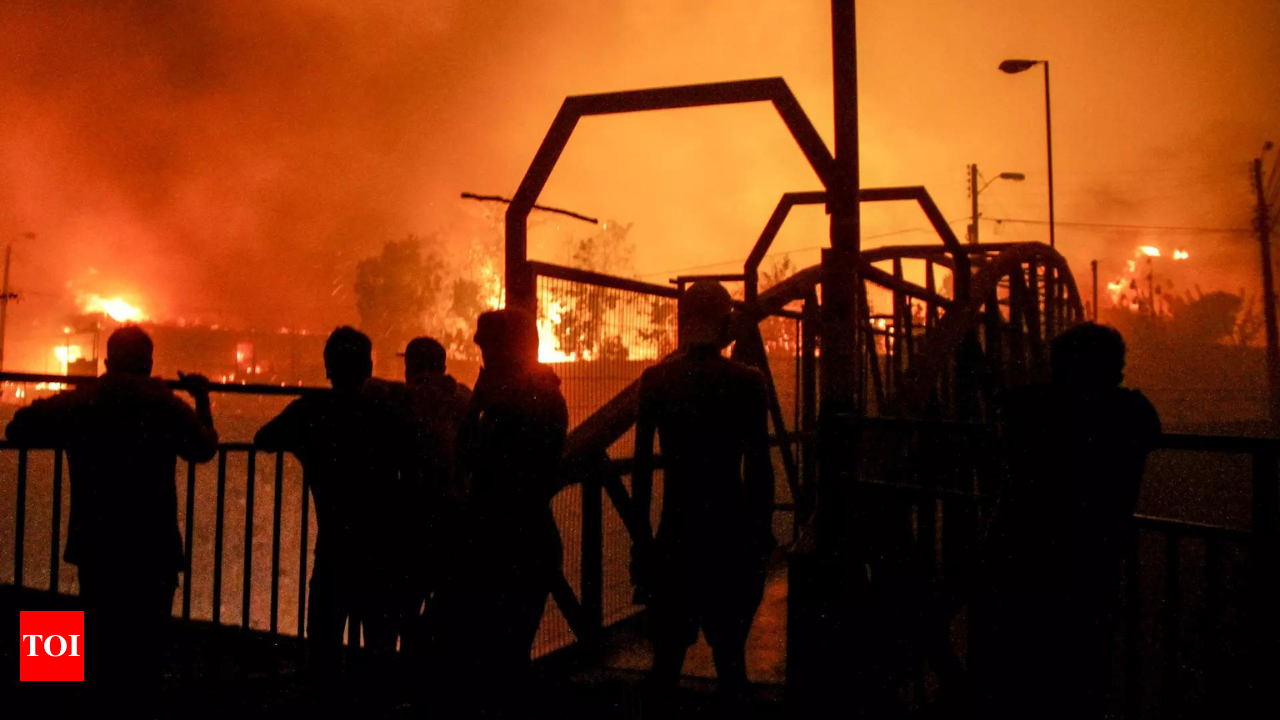In this intense and dramatic scene, a group of silhouetted individuals stand on the edge of a small iron footbridge, looking out over a body of darkened water towards a raging inferno that has engulfed a town. The night sky is painted in vivid hues of orange, red, and dark brown, suffused with thick, golden-colored smoke. The bridge, characterized by its squared-off arches leading to the main archway, frames the chaotic backdrop of buildings and trees consumed by flames. In the bottom left corner of the image, a red square with "TOI" in white text identifies this as a journalistic photograph. The figures' identities are obscured by the shadows and the overwhelming brightness of the fire, capturing a moment of shared horror and helplessness.